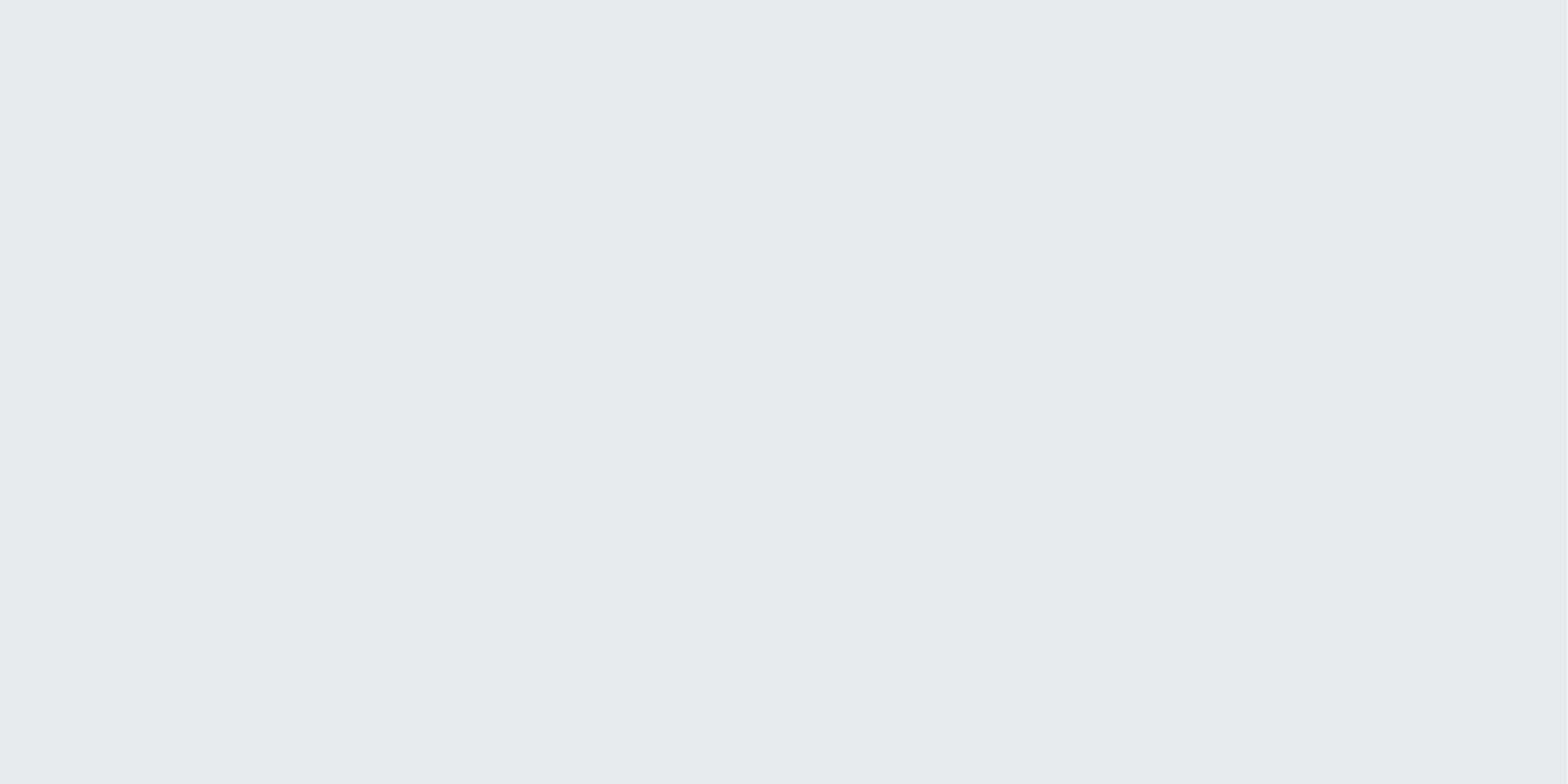The image depicts a light gray rectangle with no prints, images, or graphics. The color gradient shifts subtly from a lighter shade of gray on the left to a slightly darker shade toward the bottom right. The rectangle features a horizontal orientation, being longer on the top and bottom edges, which are of equal length, while the vertical sides are shorter but also equal to each other. The rectangle appears neither overly thin nor thick, measuring a few inches in both length and width. Beneath the gray rectangle, a plain white background extends without any text or additional elements.